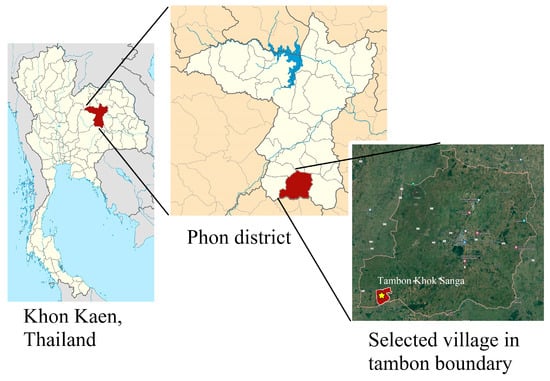The image features a series of three maps of Thailand, emphasizing a hierarchical relationship between different geographic levels. The leftmost map displays a detailed, labeled map of Thailand with a specific focus on the Khon Kaen province, highlighted in red. The central map is an enlargement of a section of the first map, pinpointing the Phon District within Khon Kaen, also marked in red. The rightmost map provides a finer, realistic satellite view of the terrain, zeroing in further to showcase a selected village within the Tambon Kok Senga boundary. Black lines connect these maps, visually demonstrating how each map segment zooms into a more detailed area within the previous map, establishing a clear relationship between the broader region of Thailand, the subdivision of Khon Kaen, and the specific localities of the Phon District and Tambon Kok Senga. The image also depicts a large body of water located to the north of the Phon District, emphasizing key geographical features in each inset.